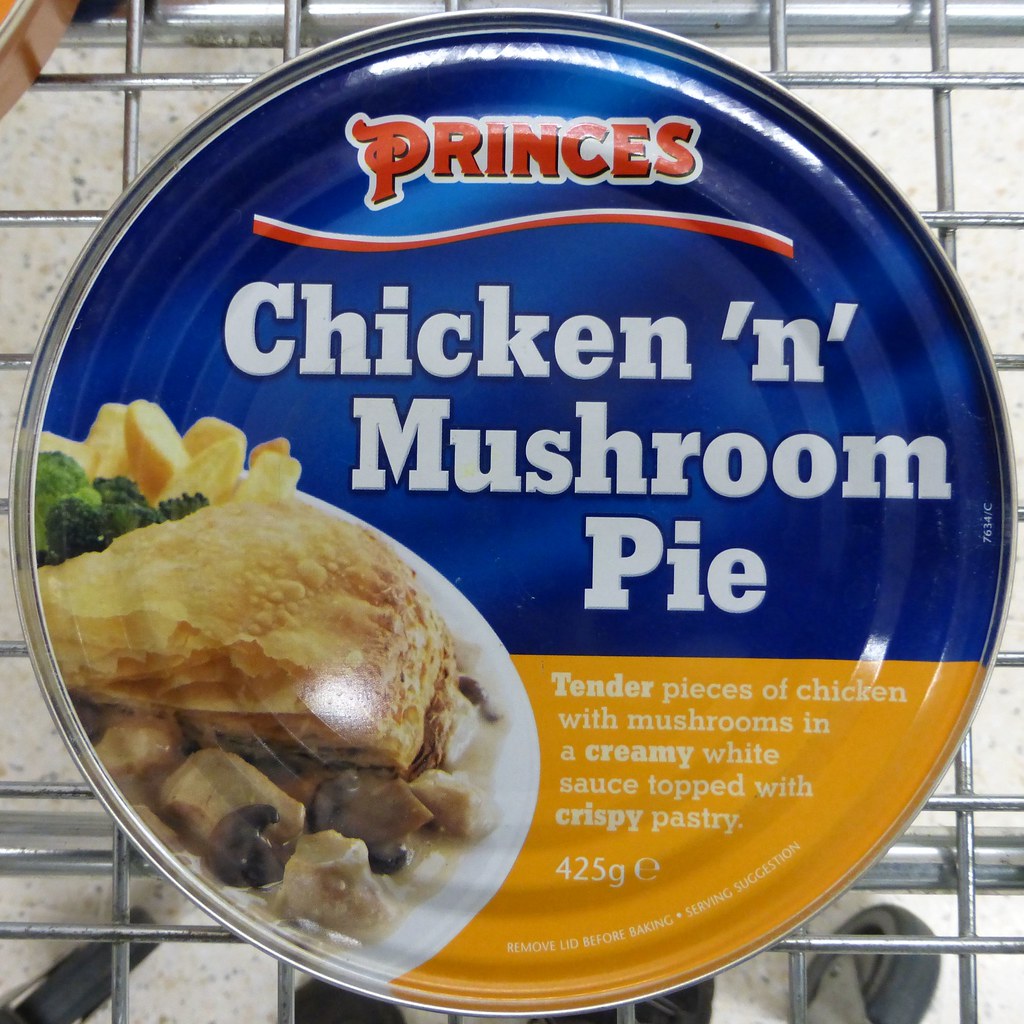This image showcases a curious culinary creation: a chicken and mushroom pie packaged in a distinctly wide can, approximately 8-10 inches in diameter. Captured from an overhead perspective, the photograph reveals the can resting on a metal baking rack, presumably prepped for the oven. The can is a perfect circle, with its upper half in bright cobalt blue and the lower half in vivid yellow. The brand name "PRINCES" is prominently displayed at the top in bold red letters, heavily outlined in white, accompanied by a swoosh design that adds a dynamic visual element.

The label clearly reads "CHICKEN 'N' MUSHROOM PIE" in striking white text against the cobalt blue background, with further elaboration on the yellow half: "Tender pieces of chicken with mushrooms in a creamy white sauce topped with crispy pastry." Below this description, the label specifies "425g" and includes a trademark or copyright mark. Adjacent to the text, there's a photograph depicting the fully prepared dish on a white round plate, showcasing the delectably baked, golden-brown pie crust.

This ready-to-bake packaged meal, unfamiliar to typical American cuisine, stands out both for its packaging design and the promise of a savory, comforting meal. The instructions suggest removing the lid before baking, making it a convenient and visually striking product for those seeking an easy, yet indulgent dinner option.